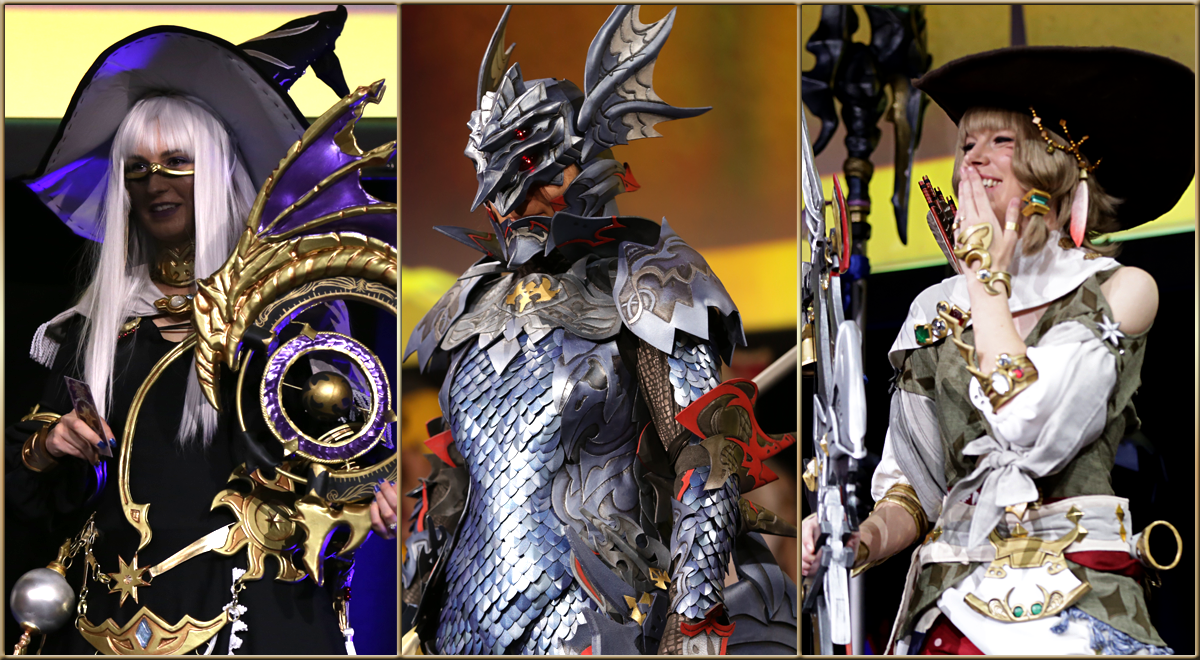This three-panel landscape image seems to capture a vibrant array of fantasy costumes, likely taken at a Comic-Con event. The left panel features a woman dressed as a witch, adorned with a black hat, long white wig, and gold-rimmed glasses. She wears a dark, possibly navy blue or black robe with intricate gold embellishments and holds a gold shield with a central purple circle surrounding a globe. Additionally, there is a bright, shiny silver orb with two gold handles and a crowned base in the bottom left corner of her panel. 

The middle panel showcases a figure clad in striking silver armor, possibly depicting an aquatic or reptilian character. This individual sports a silver helmet with wing-like extensions that transition to cream and red at the tips. Their breastplate and arms are covered in detailed silver metalwork, with a prominent gold badge on the chest.

In the right panel, a light-skinned woman appears dressed in pirate-inspired attire. She wears a black hat adorned with brown beads and a pink feather, has blonde pigtails held together with green gems surrounded by gold, and large, shapely gold bracelets on her wrist and upper arm. Her outfit consists of a light brown dress exposing her left shoulder. She holds a silver tool in her right hand, adding to her eclectic and exotic look.